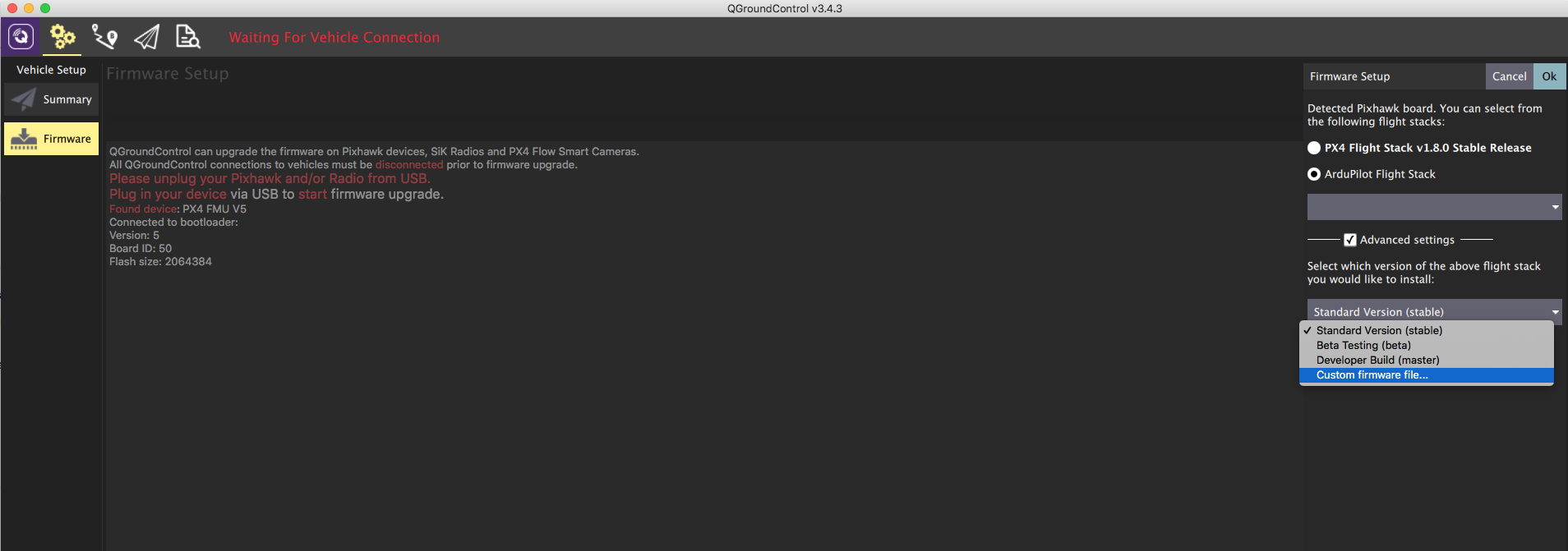The image is a screenshot of a section of a settings panel from Q Ground Control version 3.4.3. At the top center, it features the version information on a thin, light gray banner. In the upper left corner of this banner, there are three colored dots: red, yellow, and green. Directly below, there's a dark gray header bar with five icons arranged vertically on the left side. The first icon is a purple box, followed by three small, light yellow gears, underlined with a yellow line, indicating the current active screen. The next three icons are white, and to their right, red text reads "Waiting for Vehicle Connection."

On the left side of the screen, a sidebar highlights "Firmware" in light yellow. In the top left corner of a large gray background area, very small white and red text is visible. On the right side, there's a dropdown column labeled "Firmware Setup," with "Cancel" and "OK" buttons beneath. The main text indicates the ArduPilot Flight Stack, highlighted in a box. Below, two small gray headers are present, with the lower one expanded via a scrollbar. The "Standard version" option is checked, and "custom firmware" is highlighted with a thin blue horizontal strip.